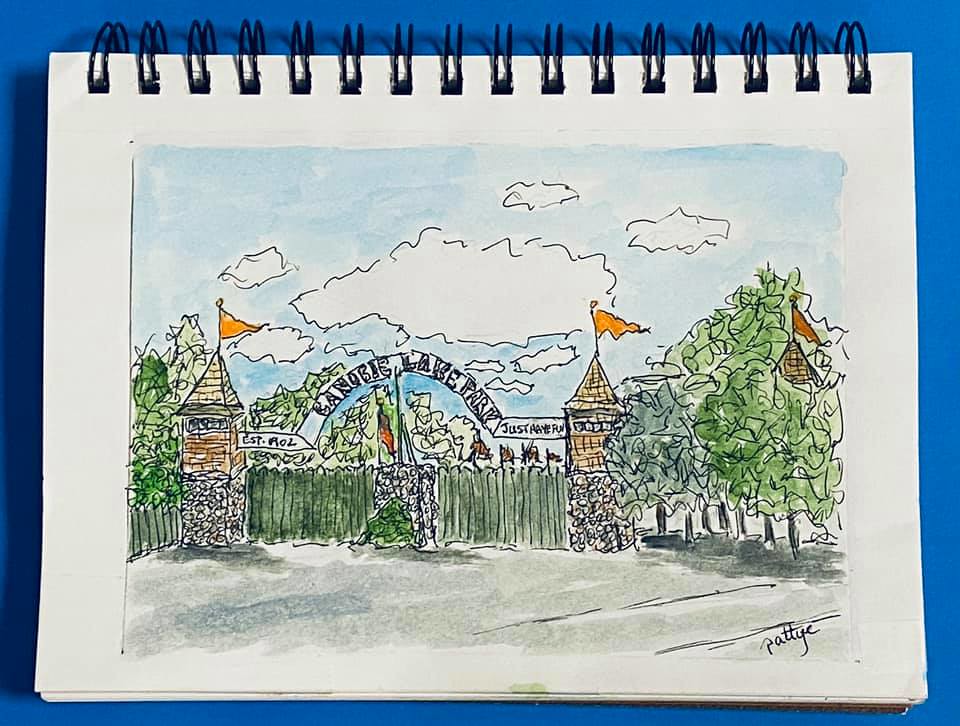In this vibrant and meticulously crafted drawing set against a serene blue background, we are presented with a whimsical depiction of an amusement park. At the heart of the illustration stand two tall brownstone towers, adorned with cheerful orange flags fluttering atop. Between these towers lies an inviting gated area, lush with greenery, enhancing the scene's enchanting ambiance. In front of the towers, a semi-circular archway bears an inscription, though its exact wording is difficult to decipher. Above the scene stretches a bright blue sky, dotted with fluffy white clouds, adding to the overall charm and sense of wonder. Notably, the artwork is signed by the artist, "Pattye," in the lower right corner, marking it as a piece created with human touch and creativity.